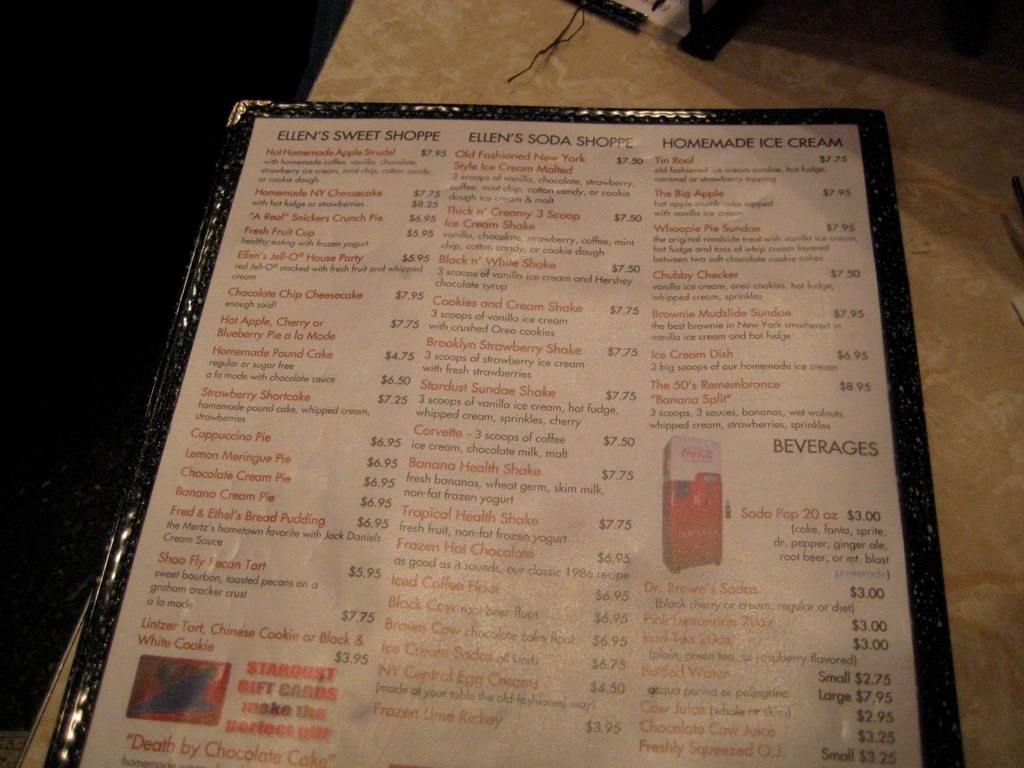A low-resolution, amateur photo taken in a dimly lit restaurant named Ellen's Sweet Shop captures a vintage-style menu placed on a table. The menu, though somewhat blurry and partially cropped out of the frame, is the central focus of the image. It appears to be enclosed in a laminated plastic sleeve with a black trim edged in chrome, attempting to add a touch of elegance that seems unconvincing. The menu lists various desserts, including "Jell-O House Party," strawberry shortcake, and cappuccino pie, alongside prices. It also features options for ice cream floats made with soda, indicating that Ellen's Sweet Shop specializes in sweet treats and desserts. The overall atmosphere suggested by the image is nostalgic but lacks clarity due to poor lighting and focus.